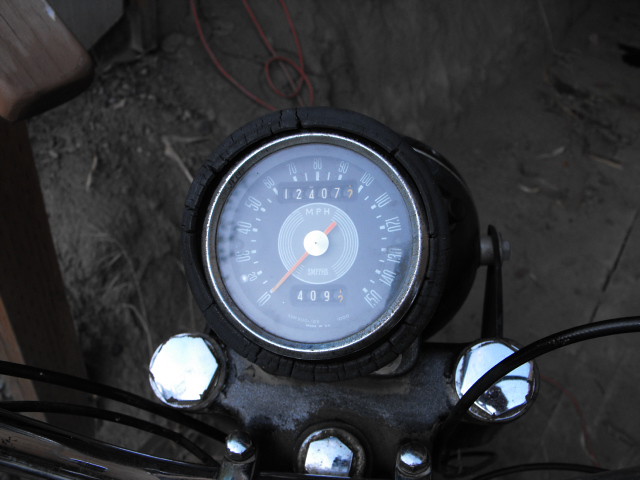This photograph captures a close-up view of a motorcycle's speedometer gauge. The black circular gauge, surrounded by a time-worn and weather-cracked casing, is the focal point. Three large bolts and two smaller bolts are also visible, securing the gauge in place. Black wires snake across the scene, likely originating from the handlebars and leading down to the brakes. 

The speedometer's range starts at 10 mph and goes up to 150 mph, with numbers marked by tens in white text. The orange needle stands at the 10 mph mark. At the center of the gauge, a gray circle bears the "MPH" label in white letters, accompanied by an unreadable word beneath it.

Above the central circle, an odometer displays a reading of "12407" in white text, followed by an orange number "5". Below this, a trip meter shows "409" in white numbers, with an orange decimal figure midway between 1 and 2.

In the background, the ground is visible with concrete and some dirt scattered at the edges. An orange electrical cord and part of a brown wooden chair arm subtly appear in the scene, adding context to the setting.